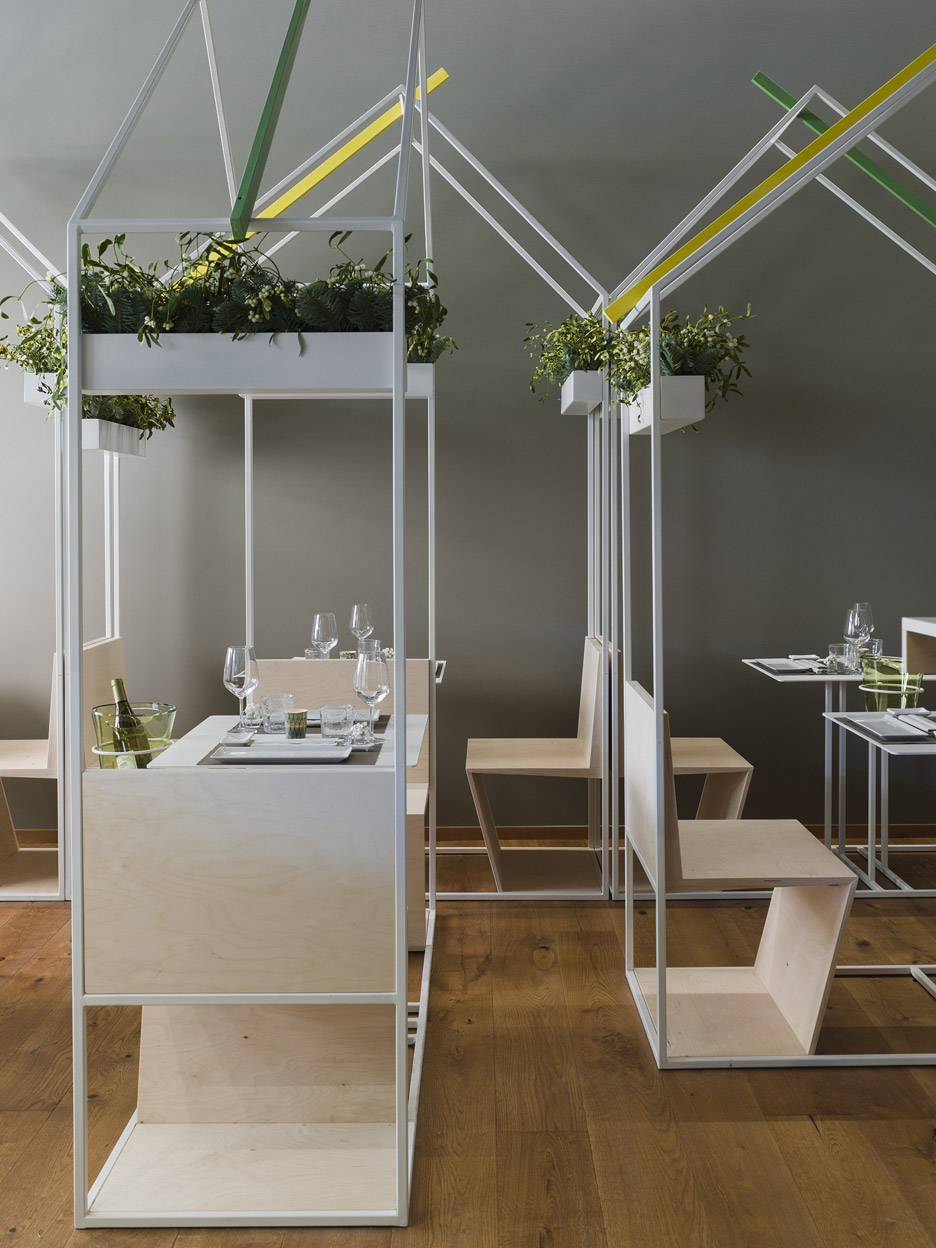The image showcases a striking white structure adorned with elegant white planters positioned at the top. Below, there is an arrangement of beige wood-colored chairs on either side of pristine white tables, each table set with clear glassware. On the left side of the table, a light green, glassy bucket adds a touch of color to the scene. Additionally, the top part of the image features green and yellow poles, casting subtle shadows on the wall behind, creating an interplay of light and shadow.